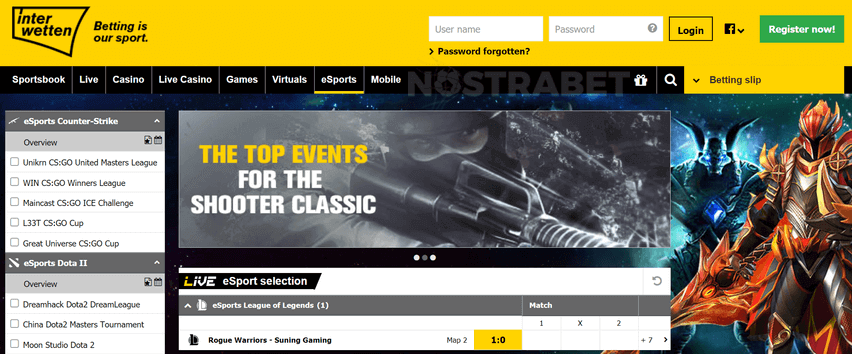The image is a promotional banner for the sports betting website Interwetten, characterized by its distinctive black and yellow color scheme. Dominating the top of the page is a vibrant yellow banner featuring the black Interwetten logo, accompanied by the slogan "Betting is our sport" prominently displayed in black text. In the upper left corner, there are input fields with white backgrounds where users can enter their username and password, accompanied by a yellow and black login button. Below these fields, a clickable text labeled "Password forgotten" with an adjacent arrow suggests a drop-down menu for password recovery options. A Facebook icon, also equipped with a drop-down arrow, hints at additional social media login options.

In the upper right corner, a standout green button with "Register now" written in white invites new users to create an account. Directly below this, a black navigation bar features options such as Sportsbook, Live Casino, Live Casino Games, Virtuals, E-sports, and Mobile. The E-sports tab is highlighted with a yellow underline, indicating it is the current selection.

The main content area is filled with eye-catching banners relating to E-sports. One prominent banner showcases an image of a knight clad in stylized red armor beside a fantastical creature, setting a dramatic tone. Another large banner advertises top events for the "Shooter Classic" and displays an assault rifle, hinting at a Counter-Strike theme with a character in a helmet and mask. Beneath this, a visible betting entry allows users to wager on a specific League of Legends match, enhancing the site's focus on diverse E-sports betting opportunities.